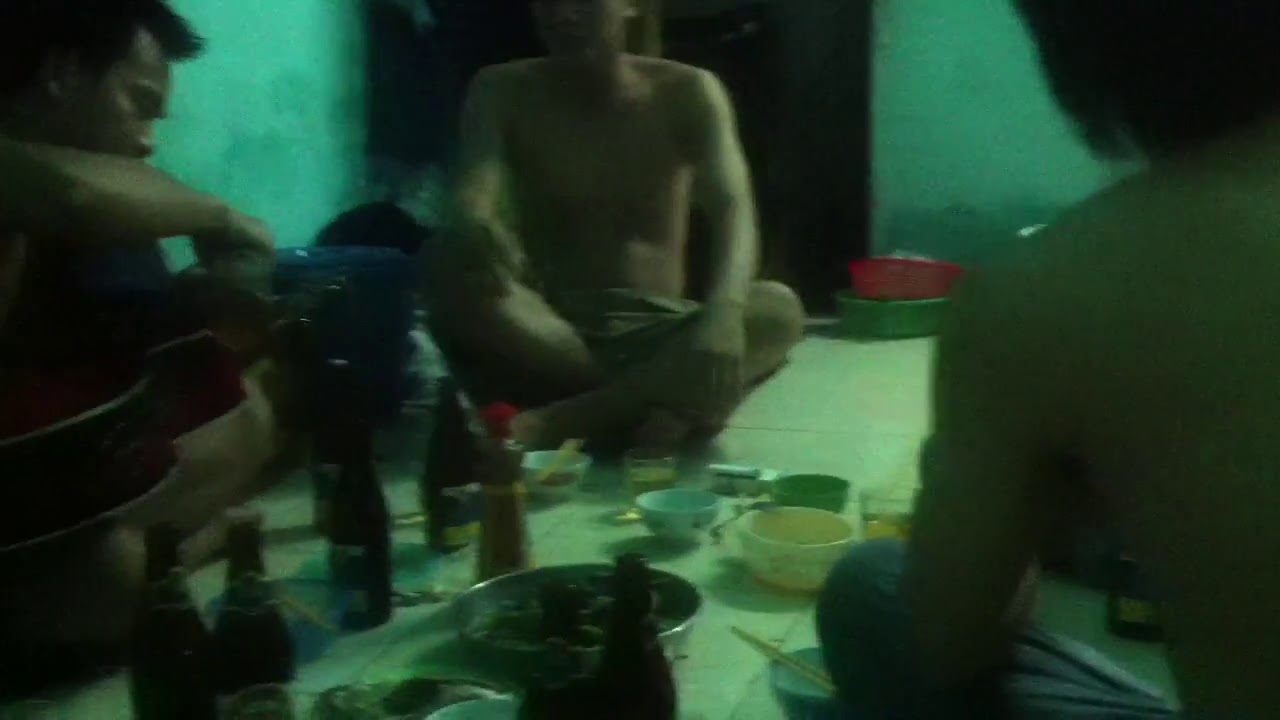In a dimly lit, blurry photograph, a group of three shirtless men, except for one man in a sleeveless black shirt on the left, are seated on the ground in a sparse room. The man on the left appears to be holding and possibly playing a guitar. The other two men, with bare upper bodies, are sitting cross-legged, with one in khaki pants and the other with blue pants. Scattered around them on the floor are a variety of items including plates, bowls, and an assortment of bottles, likely beer bottles given their dark brown color. At the center of their gathering is a large silver plate containing a dark food. Other notable items include a cylindrical sauce bottle with a red cap and a bowl with chopsticks. The men are positioned as if they are engaging in a communal meal, surrounded by the disordered array of their dining implements.